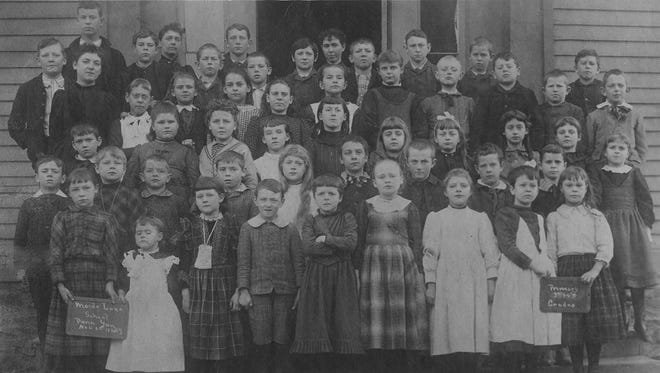The image is an old black-and-white photograph capturing a class of young Caucasian children posed in front of a schoolhouse. The children are arranged across several rows, with the tallest children likely standing on stairs at the back, making them appear elevated. A single adult, positioned third from the top on the left side, oversees the group. The backdrop features a building with distinctive clapboard siding and a centrally located doorway, dark and unadorned.

In the front row, two children stand out as they display signs, one at the bottom left and the other at the bottom right. The girls in the photo are dressed in either white or gray dresses, while the boys sport formal attire, including jackets and knickers or pants. The overall attire of both the boys and girls suggests a formal setting typical of a school photo from the early 1900s. The image conveys a sense of historical formality and simplicity, marked by the monochromatic palette and the traditional school setting.